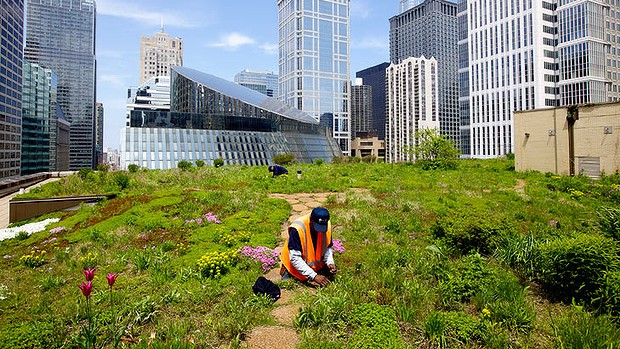In an urban setting reminiscent of the New York skyline, characterized by a mixture of high-rise skyscrapers—some made entirely of glass, others with concrete facades, and a few boasting unique architectural designs like cylindrical shapes cut at an angle—an outdoor photograph captures a tranquil rooftop garden contrasting the bustling city below. Dominating the scene, the garden features expansive green spaces interspersed with vibrant flowers such as pink tulips and yellow dandelions, alongside an array of green bushes. A stone pathway winds gracefully through this green oasis. Central to the image is a man clad in an orange construction jacket with long sleeves and a dark hat, kneeling amidst the flora. He appears to be diligently tending to the plants, perhaps pulling weeds or planting new growth. Another individual, dressed in black, can be seen in the distance, similarly engaged in gardening tasks. The photograph, taken during the day, showcases a clear blue sky peppered with thin white clouds, enhancing the serene yet industrious atmosphere of this urban rooftop retreat.